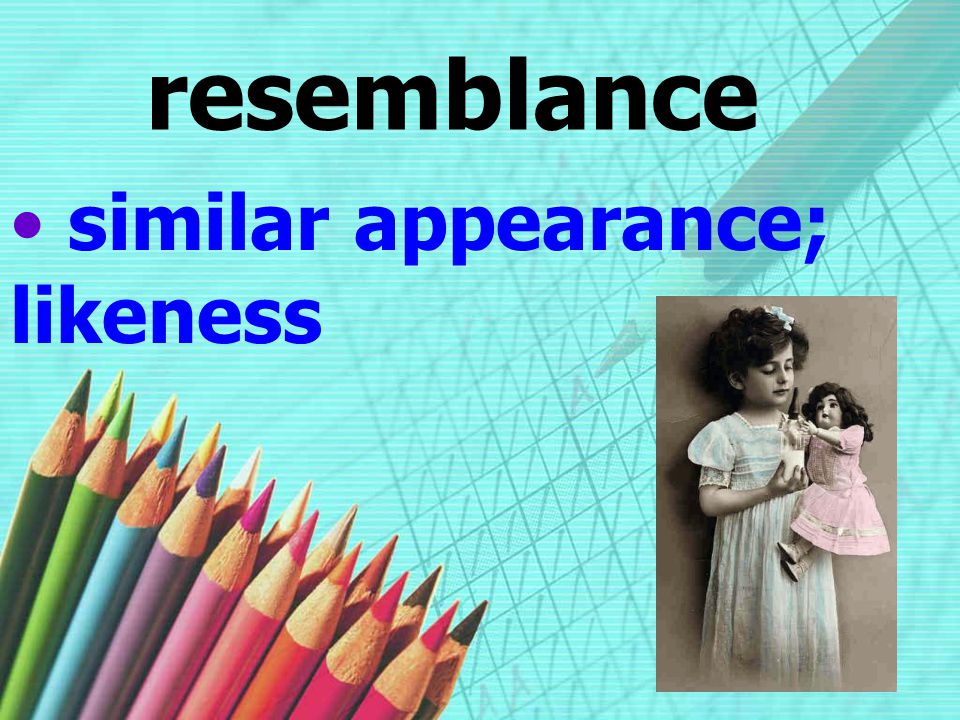The poster, entitled "Resemblance," features a collage of images set against a light blue background. At the top, "Resemblance" is written in black font, followed by "Similar Appearance" and "Likeness" in blue font, separated by a purple bullet point. Below this text, on the bottom left, are the tips of various colored pencils in hues including green, yellow, blue, purple, pink, orange, and red. To the right of the pencils, there is a photograph of a young girl wearing a white dress, holding a doll in a pink dress, highlighting their similar appearances. The background has a faint image of a pencil filling in squares on a sheet of paper, perhaps a crossword puzzle. The combination of these visual elements creates a thematic representation of resemblance and likeness.